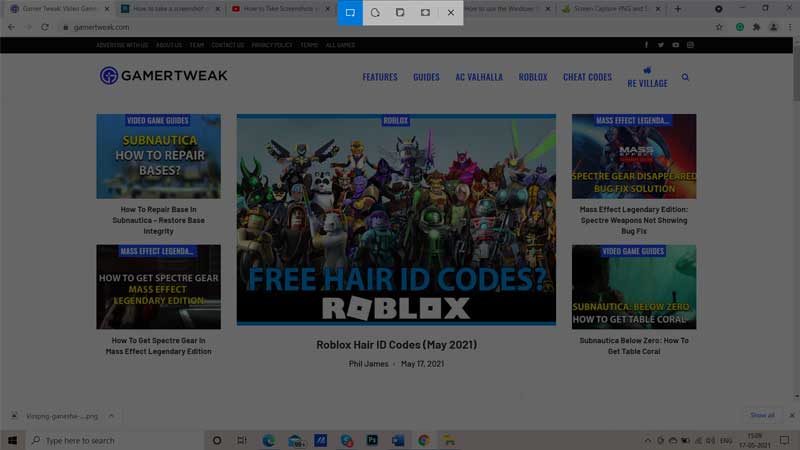**Caption:**

The image is a landscape-format screenshot depicting a browser window with a pop-up overlay. The overall tone is darkened due to the active pop-up.

**Browser Interface:**
- **Tabs**: At the top left, there are six open tabs, each with an indistinct title and corresponding icon. To the right of these tabs is a plus sign for opening new tabs.
- **Window Controls**: In the top right corner, we see the standard window control icons: a round circle, a dash for minimizing, a restore/maximize icon, and an X for closing the window.

**Pop-Up Details:**
- The pop-up is oblong with five icons aligned horizontally. From left to right, the icons are:
  - A square (highlighted in blue).
  - A crescent moon.
  - A folder.
  - A circle within a dark square.
  - An X.

**Active Tab Content:**
- The active tab is identified as "Gamer Tweak," with a purple and white G logo.
- Across the top of the webpage, blue capitalized headers read: Features, Guides, AC Valhalla, Roblox, Cheat Codes, ReVillage, and a magnifying glass icon.

**Main Content:**
- The main section features a central image with a blue rectangle reading "Roblox" at the top. Below the image, large text reads "Free Hair ID Codes, Roblox," with "Free Hair ID Codes" in blue capitals and "Roblox" in bold, thick capitals. The first 'O' in "Roblox" is a tilted square.
- The background of this main image contains various warrior-like characters from the Roblox game, each unique in color and appearance.

**Subsection Content:**
- To the right of the main image are two smaller images:
  - The first is under a blue banner reading "Mass Effect Legendia" and includes a blue and red futuristic image with the text "MASS Spectre Gear Disappeared Bug Fix Solution."
  - The second features a green abyss with a blue banner titled "Video Game Guides," containing the text "Subnautica Below Zero" in yellow, and "How to Get Table Coral" in white.

**Intervening Text Sections:**
- Between these two images:
  - Text reads "Mass Effect Legendary Edition Spectre Weapons Not Showing Bug Fix."
- Below the second image:
  - Another text snippet "Subnautica Below Zero How to Get Table Coral."

**Additional Images on the Left:**
- Two images mirror the layout on the right:
  - The first is under a blue banner reading "Video Game Guides," with a cartoonish ship and the text "Subnautica in yellow, How to Repair Bases in white."
  - The second is under a blue banner "Mass Effect Legend Agenda" with the text "Mass Effect Legendary Edition in yellow, How to Get Spectre Gear in white."

**Footer and Browser Bar:**
- At the very bottom, the Windows taskbar is displayed with the following:
  - A Windows icon at the bottom left corner.
  - A search bar labeled "type here to search."
  - Seven or eight icons, including a globe, an envelope, a blue square with white dashes, the Google Chrome logo, and a folder.
  - A share icon in the bottom right along with other indecipherable icons.
  - Text reading "ENG," the date "1705, 2021," and the time "15:20."